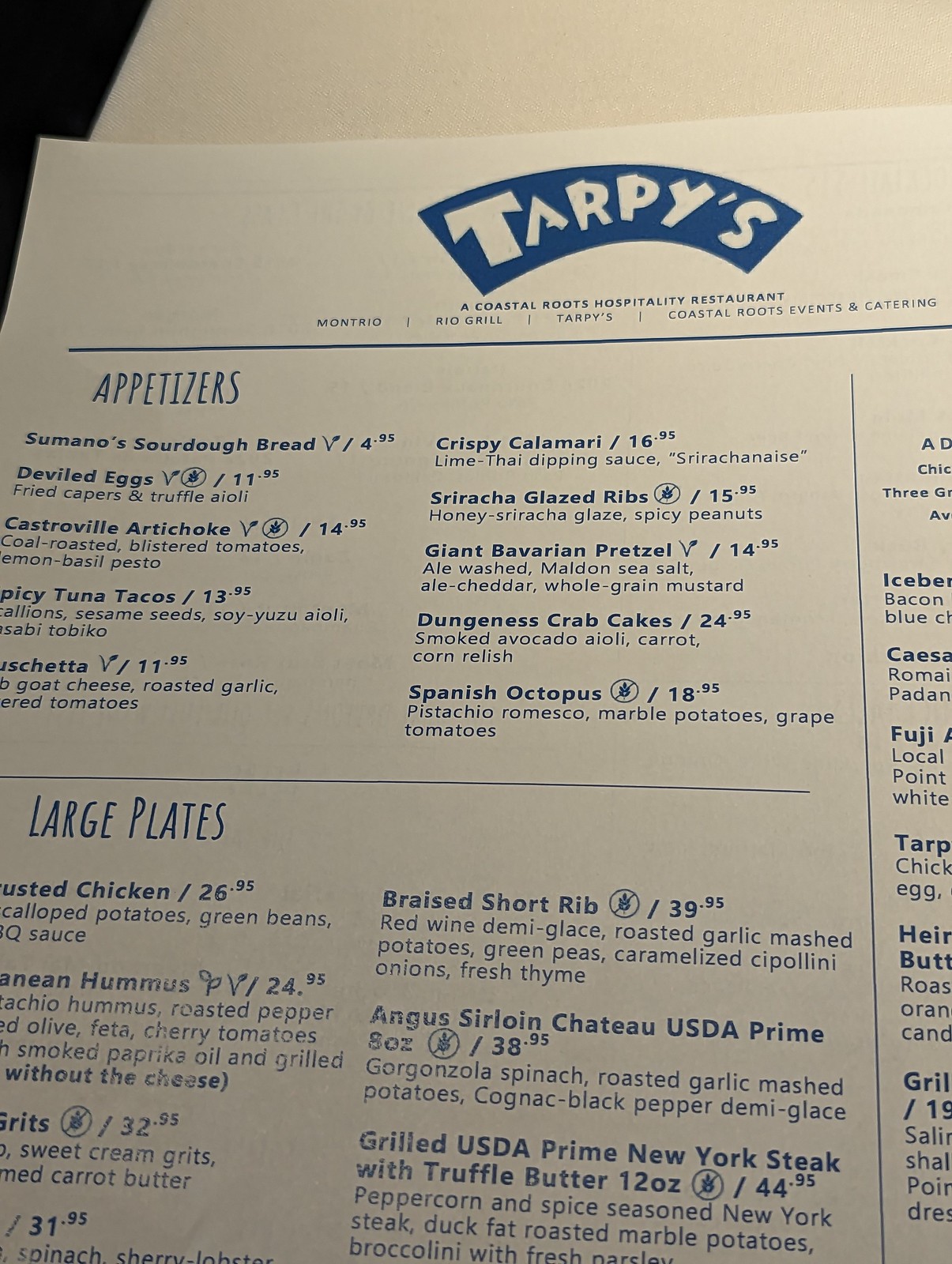The image depicts a menu from the restaurant Tarpy's, prominently displayed against a white table. The menu itself is a large white sheet with dark blue font. The title "Tarpy's" is positioned at the top in a thick, kooky, arc-shaped font against a navy blue color block also in an arc formation. Beneath the title, the words "A Coastal Roots Hospitality Restaurant" are printed in small all-capital letters, followed by the names of associated establishments: Montreal, Rio Grill, Tarpy's, and Coastal Roots Events and Catering.

A thicker horizontal line separates the top section from the rest of the menu, where two main categories, "Appetizers" and "Large Plates," are written in a tall, thin, handwritten font reminiscent of marketing for certain trendy products. Items listed under "Appetizers" include castro artichokes, spicy tuna tacos, Spanish octopus, and a giant Bavarian pretzel. The "Large Plates" section features options like braised short rib, chateau sirloin, prime steak, and Mediterranean hummus. The descriptions of these dishes are in a regular, unbolded sans serif font, while the items themselves are in bold.